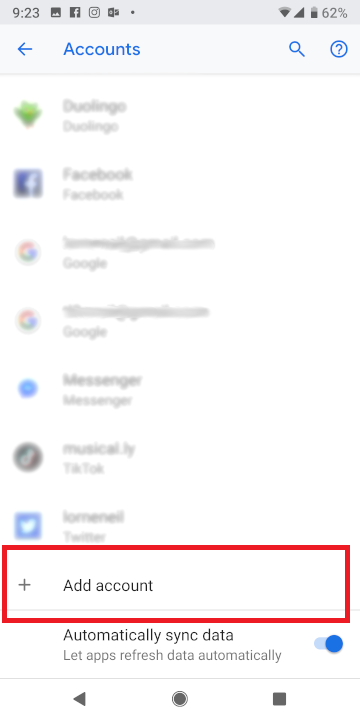Here is a cleaner and more detailed descriptive caption for the image:

---

This screenshot, taken from an Android phone or tablet, depicts various notifications and interface elements. At the top of the screen, the time is displayed as 9:23. A series of notifications follow, including a screenshot notification, a Facebook notification, an Instagram notification, and a Windows notification. 

On the right-hand side of the status bar, icons indicate the device’s connectivity and battery status. The Wi-Fi signal is shown at three-quarters strength, the cellular signal is at full strength, and the battery icon displays 62%, indicating it is over half full.

Below the status bar, a lighter gray bezel with blue accents contains various navigation elements. On the left-hand side, there's a blue arrow icon next to the word "Accounts," followed by a blue magnifying glass icon for search and a blue circle with a question mark for help.

The main part of the screen presents a list of applications, some of which are blurred for privacy. The visible apps include:
- Duolingo, identified by its green owl mascot with a yellow beak.
- Facebook, represented by a blue square with a white "F" in the center.
- Two Google accounts, each marked by the Google logo consisting of the colors red, yellow, green, and blue in the shape of a "G."
- Facebook Messenger, shown as a blue circle with a squiggle within it.
- A TikTok app icon, described as a black circle with an oblong, stylized "T," labeled as musically.ella.
- Twitter, depicted as a blue square with a white bird (Tweety) in the center.

At the bottom of the screen is a red rectangle encasing a white section that reads "Add account." Below this, there's an option labeled "Automatically sync data," with a gray description underneath that says "Let apps refresh data automatically." This option is accompanied by a blue slider. Finally, at the very bottom, standard Android navigation icons are visible: a left-pointing arrow, a circle, and a square.

---